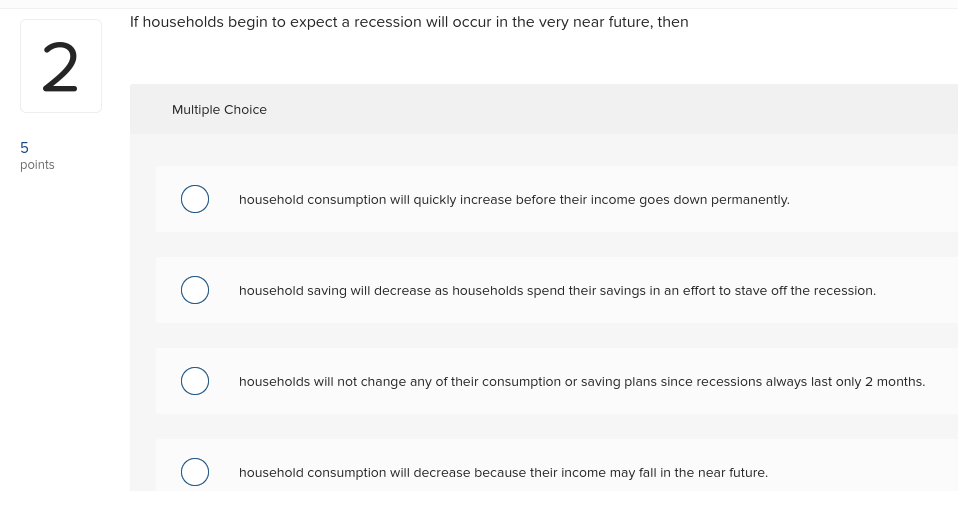Screenshot of an online quiz or survey with a clean and minimalist design. The background is predominantly white with black text, and the layout features tables in varying shades of gray to distinctly separate the different options. Displayed on the screen is question number two, which is identified as being worth five points. The question reads: "If households begin to expect a recession will occur in the very near future then," followed by multiple choice options. 

The visible options for answering the question are:
1. Household consumption will quickly increase before their income goes down permanently.
2. Household savings will decrease as the household spends their savings in an effort to stave off the recession.
3. Households will not change any of their consumption or saving plans since the recession always lasts only two months.
4. Household consumption will decrease because their income may fall in the near future.

The design is straightforward, using simple boxes and rows with different background colors to organize the information. The text size is relatively small, and there are large margins separating the different tables, enhancing the minimalist aesthetic.